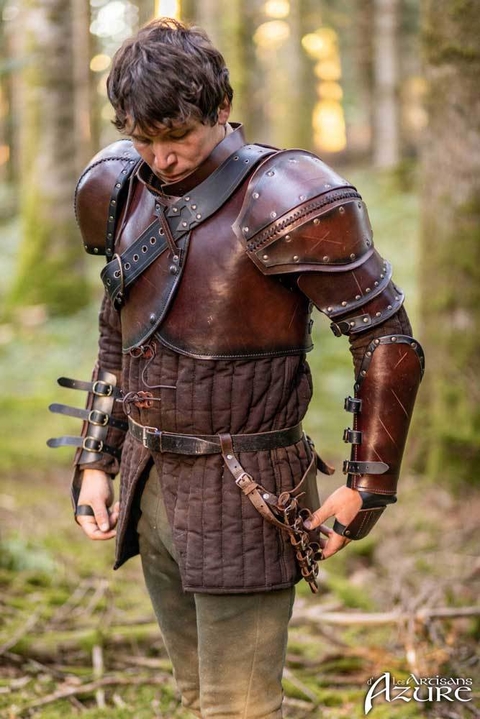In the photograph, a white male with dark hair is dressed in a detailed, old-fashioned costume, seemingly a form of bronze or dark brown leather armor. His gaze is directed downwards, adding a sense of contemplation or resolve. The costume includes a tunic and a thin leather armor adorned with assorted studs and dark brown stitching. His forearms are protected by gauntlets with multiple black leather buckles and straps, showcasing a worn, battle-hardened look. He also sports a dark brown belt with a square silver buckle, and another belt slung across his chest and shoulder. He is dressed in tight, tan or grayish leather pants, blending smoothly with the rest of his attire.

The setting appears to be a forest, bathed in daylight, with a lush, green background that is blurred to emphasize the subject. In the bottom right corner of the image, there is white text reading "Arcadian's Azure" or "Azure Artisans," suggesting a possible promotional context for the costume. The entirety of the ensemble and setting evokes a sense of lived-in authenticity, further highlighted by scratches on the armor, giving it a well-used, realistic appearance.